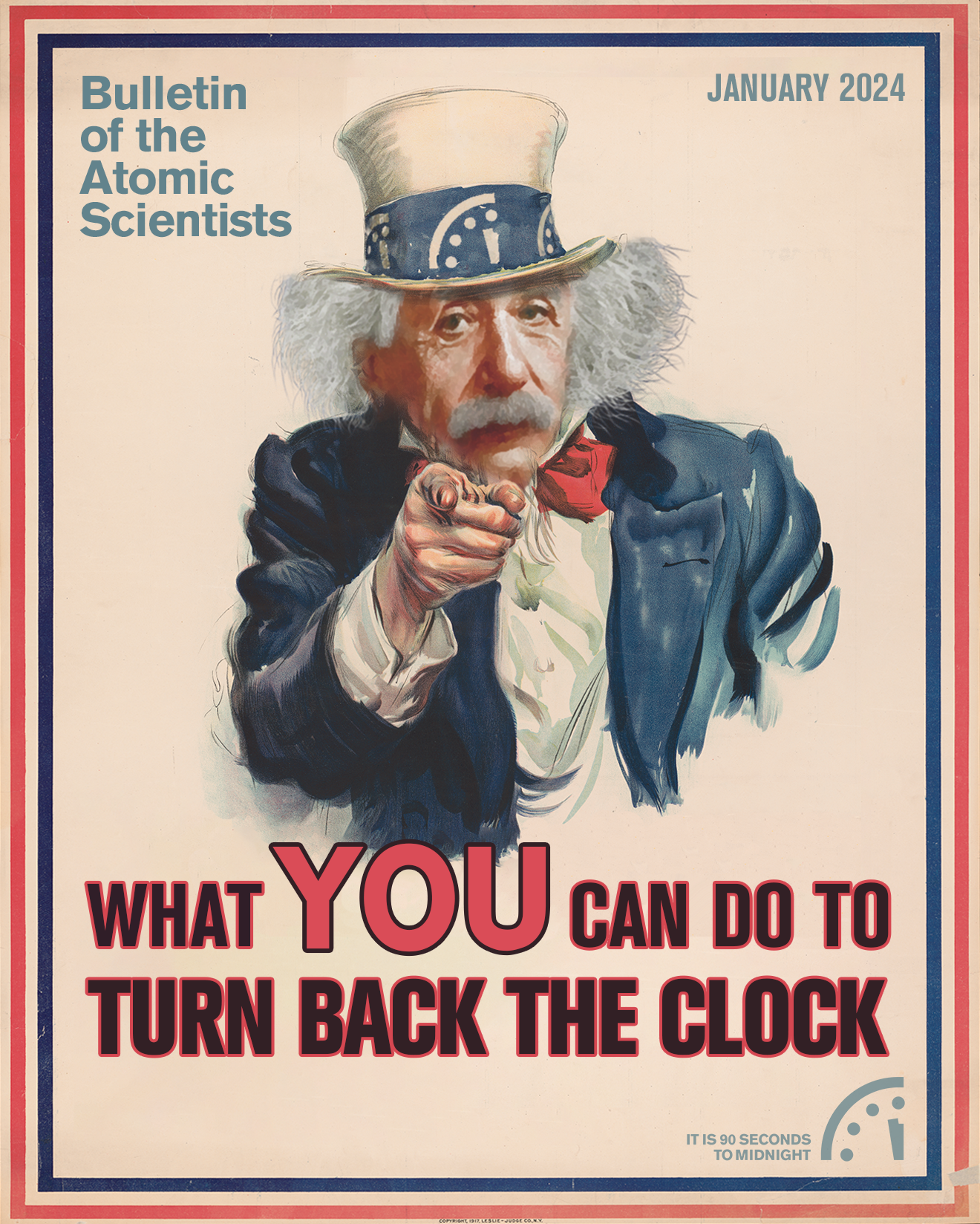The poster, set against a salmon-pink background, is bordered by dark blue lines and encased in a red frame. It features a striking, sketch-style illustration resembling the famous Uncle Sam recruitment poster, but with Albert Einstein's face. Einstein, wearing a blue suit coat, a red bow tie, and a white hat featuring a partial clock design, points directly at the viewer. Prominent text reads "Bulletin of the Atomic Scientists" in blue at the top left corner and "January 2024" on the right. Below Einstein is the bold, black and red statement: "What you can do to turn back the clock." In the lower right corner, red text declares "It is 90 seconds to midnight," accompanied by a small, partial clock illustration.